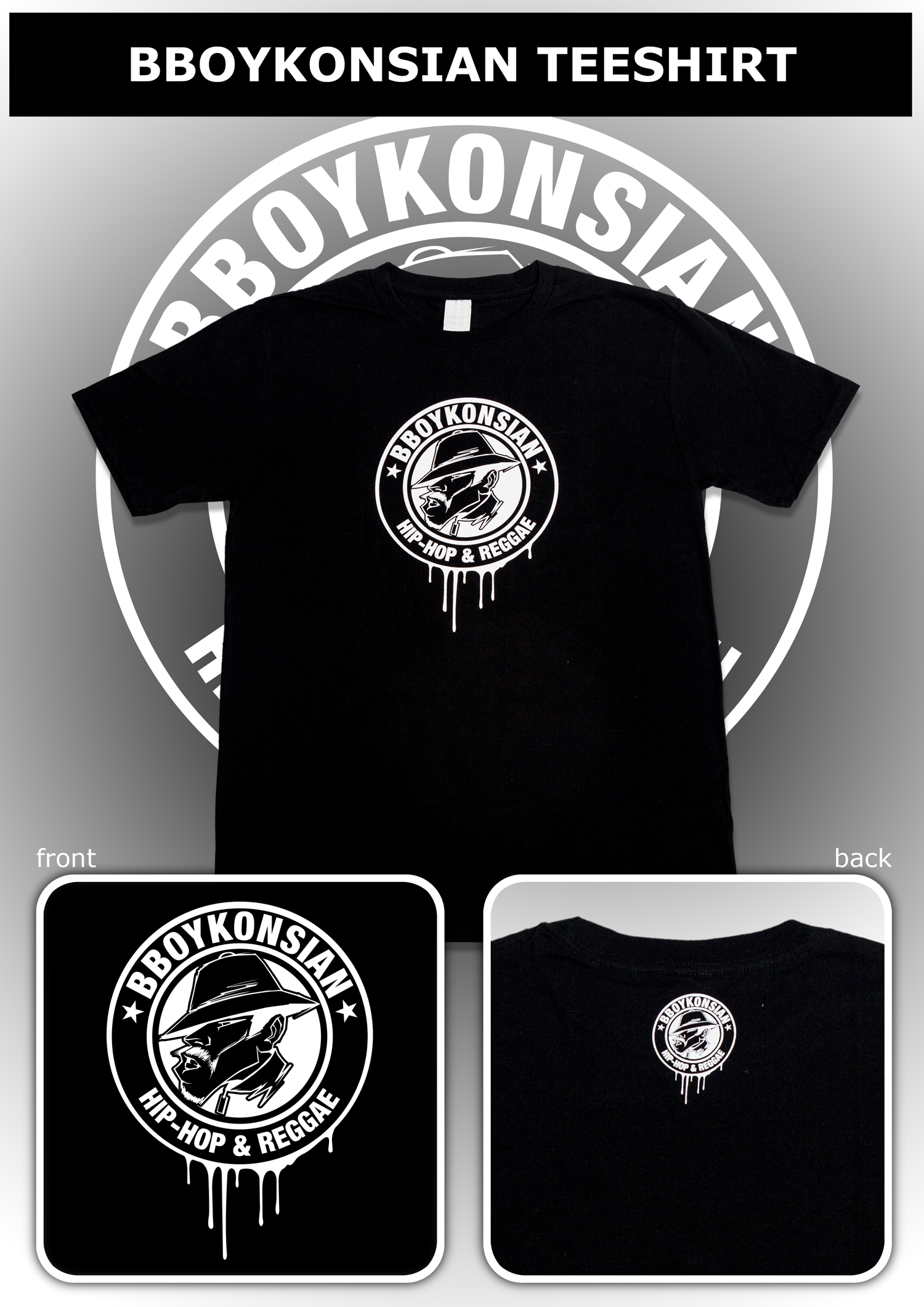The image is an advertisement for a short-sleeved black t-shirt featuring a distinctive logo. The background of the entire image fades from light gray to dark gray. At the top of the image, the title "B-BOY KANSEAN T-SHIRT" is displayed in all capital letters, in white text over a black border. The main part of the image showcases the t-shirt in the center. The t-shirt features a round logo with the text "B-BOY KANSEAN" at the top and "Hip Hop and Reggae" underneath. Inside the circle is an illustration of a long-faced figure, possibly wearing a detective's hat, with dripping paint effects beneath the circle, outlined in white. 

At the bottom of the image, two square close-ups are displayed; the one on the left shows the front of the shirt, and the one on the right shows the back. Both squares have a white outline against the gray background. The front close-up highlights the large logo from the center view, while the back close-up reveals a smaller version of the logo positioned towards the center of the neckline. The overall color scheme comprises primarily black, white, and various shades of gray. The presentation suggests this t-shirt is the product being sold.